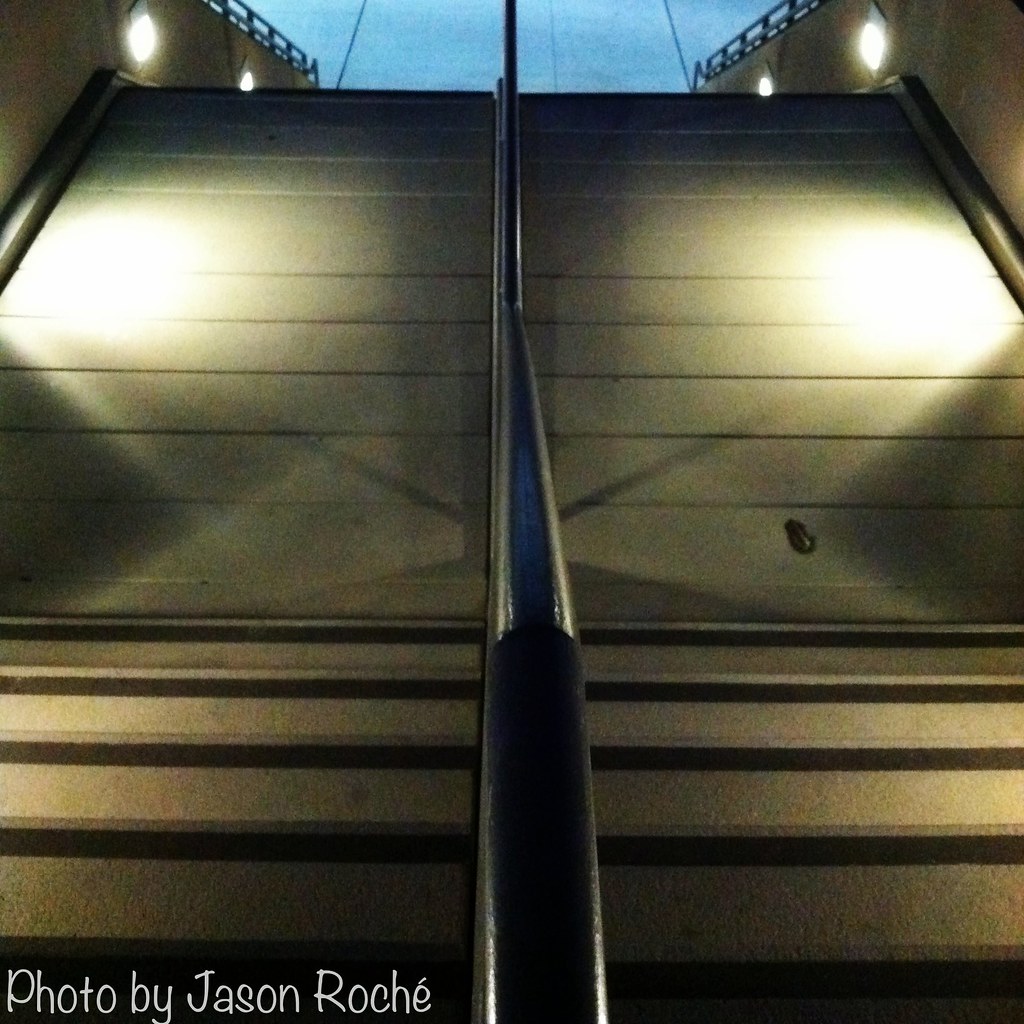This dark photograph, taken by Jason Roche and marked with his name in the bottom left corner, depicts a steep set of brownish-yellow concrete stairs, divided by a black metal handrail that casts distinct shadows across the steps. The setting appears to be a walkway or ramp, as the stairs transition from an open to a closed configuration, suggesting a movable design. The topmost steps are level, forming a flat walking surface. Lights line the sides of the concrete walls, illuminating the scene at dusk, and additional railings border the walkway on either side. Outside, visible cables contribute to the structural complexity of the image.